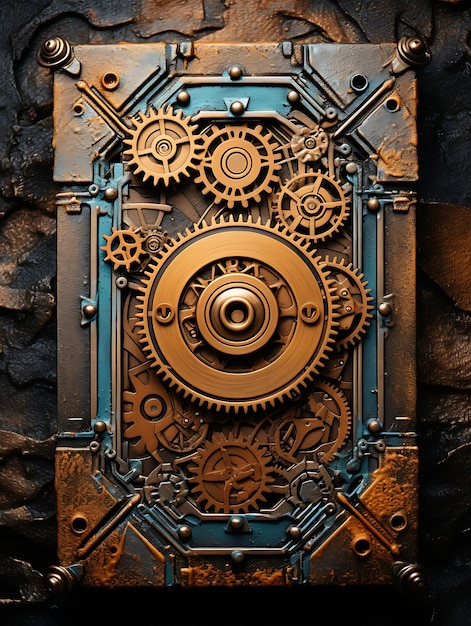The image portrays a detailed 3D art piece that emulates a mechanical contraption, reminiscent of the inner workings of a clock or a vault. The background is a blend of black and rust colors, providing a textured, metallic canvas that enhances the overall rustic aesthetic. The centerpiece of the composition is a vertically-oriented rectangular structure with knobs at each corner, giving the impression of a functional component, possibly for mounting or hanging.

At its core, the mechanism is dominated by a large golden gear encircled by smaller gears of varying sizes, all intricately arranged to convey motion and complexity. The central gear is framed by a square with each corner featuring circular protrusions. Adding a splash of color, a teal blue ring accented with bolts intersects the mechanism, suggesting a sophisticated assembly of interconnected parts.

The entire piece exudes a steampunk vibe, with its rich palette of dark gray, rust, golden brown, and accents of turquoise, inviting viewers to explore the intricacies of its design and imagine the purpose of this enigmatic, clock-like contraption.